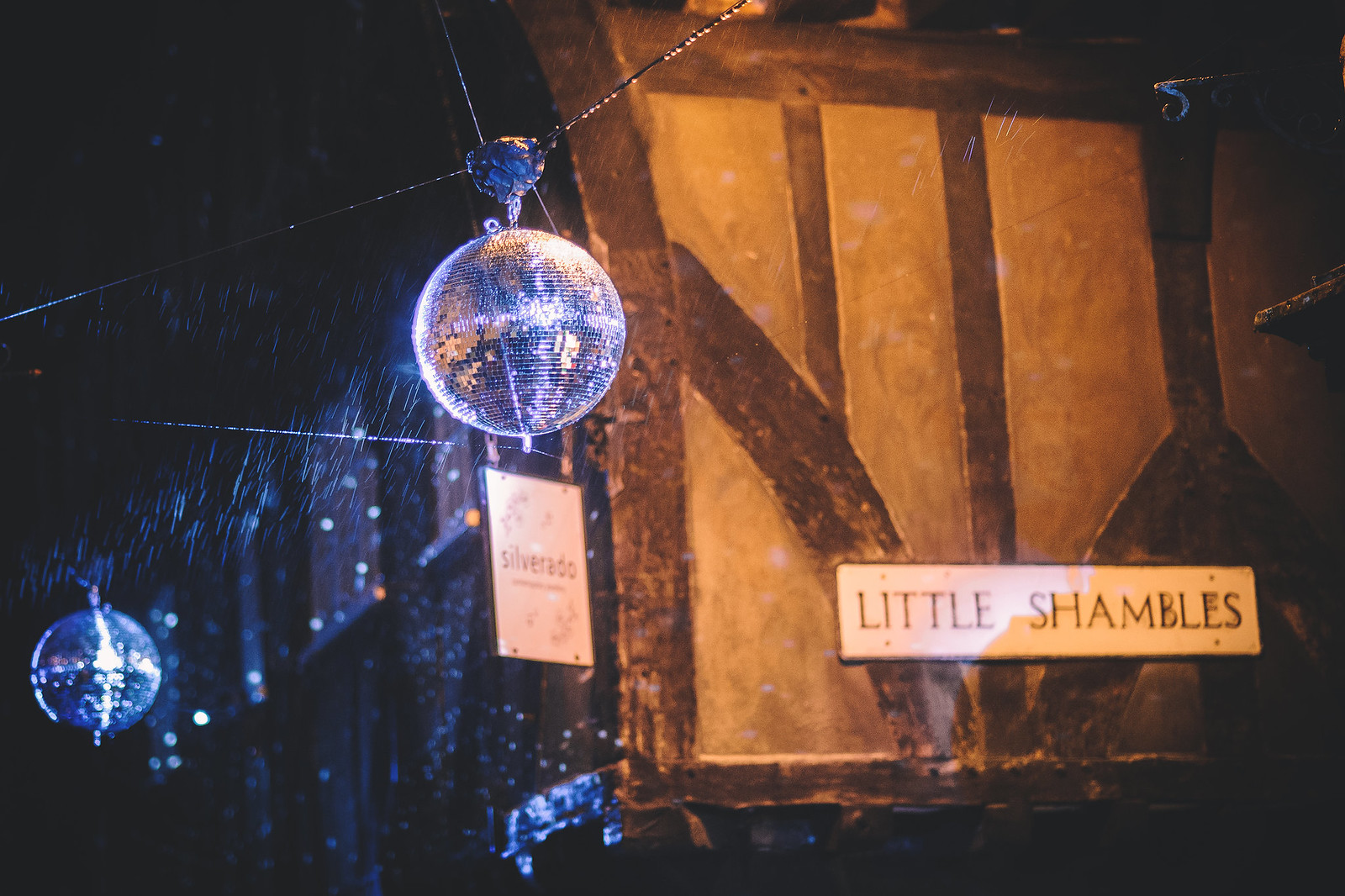In this atmospheric nighttime photograph, two glimmering disco balls hang from cables, casting specks of light in a dark setting. The scene appears to capture the exterior of an establishment, possibly a pub or club, as suggested by the signage. To the left of the image, a sign reads "Silverado," while to the right, an old-fashioned, Tudor-style sign says "Little Shambles." The backdrop features a mix of tan wooden panels and more ornate wooden designs, adding to the vintage charm of the scene. Accentuating the moody ambiance, raindrops can be seen falling, suggesting that the photograph was taken during a rainy night.